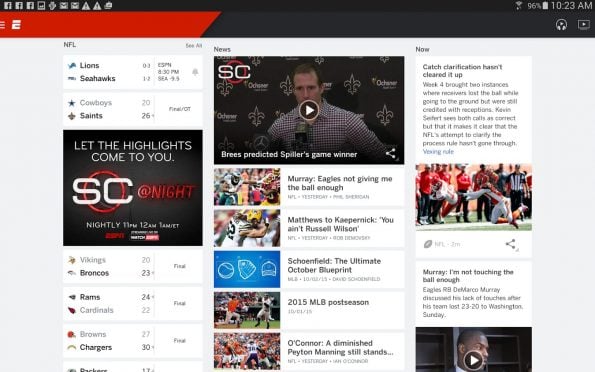The image is of a mobile website viewed in landscape mode, approximately 30-50% wider than it is tall. At the very top, a slender black bar spans the width of the screen, occupying about 5% of the height. On the upper left, there are around ten light gray icons, while the upper right displays phone status indicators like signal strength, battery life, and the time, which reads 10:23 a.m. 

Beneath this top bar, a banner occupies the upper section of the screen, with approximately the first third in red and the remaining right third in black. The main background below the banner is a light gray, hosting three distinctly labeled columns: "NFL," "News," and "Now."

In the "NFL" column on the left, scores of various games are listed. The first matchup is the Lions versus the Seahawks, followed by the Cowboys against the Saints. An advertisement appears midway down, featuring the text "Let the highlights come to you" on a black background with the logo "SC at night." Further down, more game scores are displayed: Vikings versus Broncos, Rams versus Cardinals, and Browns versus Chargers, with subsequent text cut off.

The "News" column in the center begins with a video at the top that includes play functionality. The video showcases a man behind a microphone, likely providing an analysis or synopsis of a game, possibly a coach or commentator giving his take on recent events.